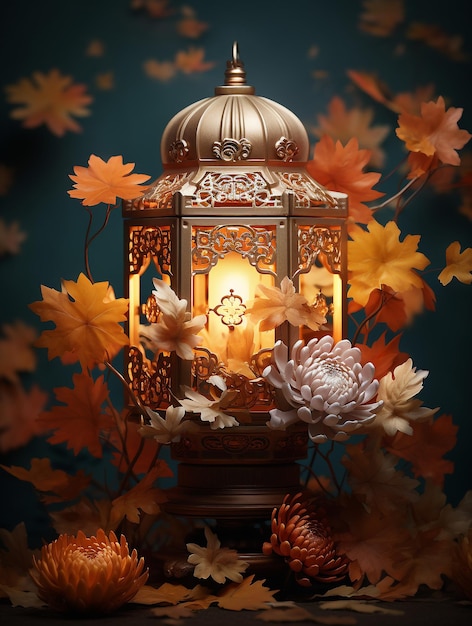This highly photorealistic, computer-generated image features an intricate, Asian-style lantern, likely made from a goldish metallic material such as brass or bronze. The lantern, which has a round, domed top with a small spire and a ring for hanging, is illuminated from within by a candle, its light visible through the glass doors encased in ornate latticework. The setting is a dark, almost navy blue background, scattered with vibrant yellow and orange leaves. The lantern rests on a surface adorned with chrysanthemums in orange and white hues, while additional leaves are spread at its base. The detailed scene includes out-of-focus flowers in the background, enhancing the depth and focus on the vividly sharp chrysanthemums in the foreground. The overall lighting appears to be influenced by an overhead source positioned to the center right of the image, creating a subtle gradient from brighter at the top to darker at the bottom, thus highlighting the lantern's ornate details and the surrounding natural elements.